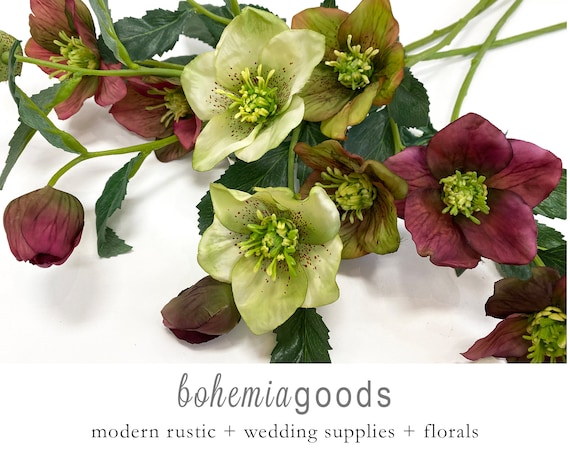The color photograph, oriented in landscape, captures a loosely arranged bouquet of Lenten Rose (Hellebore) flowers spread out on a white tablecloth, casting delicate shadows. The flowers, around eight in total, display a variety of hues: creamy white with red speckles, dull rosy red, and a compelling mix of green and red petals. Several blooms are front and center, fully open, while a few in the upper left and center left are either closed or partially opened. Each flower is attached to a light green stem adorned with sharply ridged green leaves. At the bottom of the image, the text "Bohemia" appears in cursive, followed by "goods" in a clean, non-cursive font. Below this, a smaller font reads "Modern Rustic + Wedding Supplies + Florals," suggesting the image is part of a promotional advertisement for a wedding supply company specializing in rustic and bohemian floral arrangements.